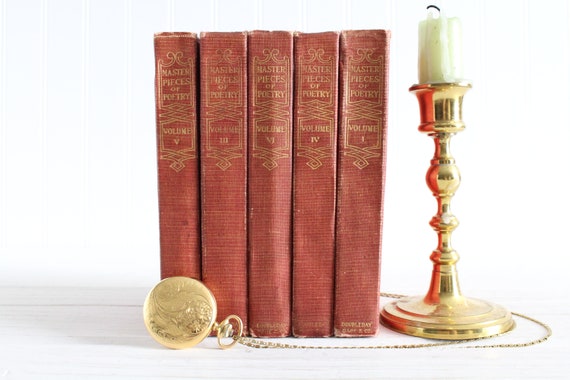The photograph, arranged in a horizontal rectangular frame, captures an elegant still-life scene featuring antique books combined with timeless objects. At the center, five distinguished books stand upright, their burgundy covers showing signs of age. Each spine bears faded gold letters, which read "Masterpieces of Poetry" with Roman numerals indicating the volumes: V, III, VI, IV, and I from left to right, suggesting some volumes are missing. Positioned to the left of the books is a tall, ornate gold candlestick with a thin middle and decorative orbs adorning its structure. The candlestick holds a short white candle that slightly exceeds the height of the books. Draped around the base of this candlestick is a gold pocket watch chain, which curves gracefully and leads to a closed pocket watch lying in front of the books. The entire arrangement rests on a white table against a plain white background, whose simplicity highlights the striking shadows cast by the books and objects, contributing to the overall vintage aesthetic.